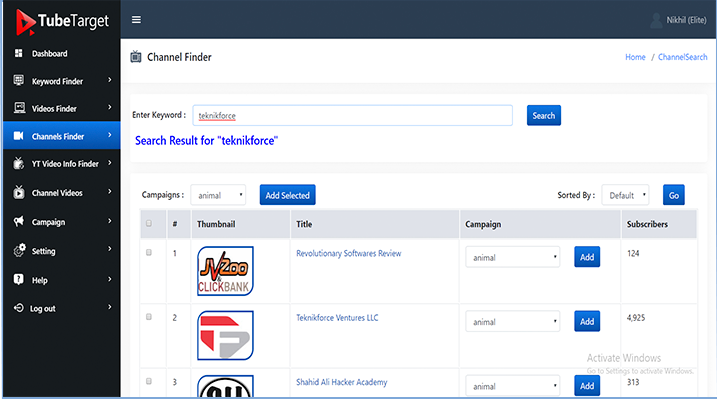The image presented is a screenshot of a web application’s interface, most likely related to YouTube channel management or keyword analysis, given the context of the elements described.

On the left side, occupying a smaller, vertical space within the horizontal frame, lies a vertical navigation menu with a black background and white text. At the top of this menu, a rightward-pointing red triangle with a smaller black triangle inside serves as an indicator. The section is titled "Tube Target." Below this heading is a list of menu options: "Dashboard," "Keyword Finder," "Videos Finder," "Channel Finder" (highlighted in blue indicating the current selection), "YT Video Info Finder," "Channel Videos," "Campaign," "Setting," "Help," and "Logout."

The larger rectangle on the right side of the image features a white background. At the top left, it says "Channel Finder" accompanied by a small TV symbol. In the upper right corner, the text appears to read "Nikhil [Elite]," although it is slightly blurry. Beneath the header, a breadcrumb navigation is displayed: "Home / Channel Search." Below this, there is an input field labeled "Enter Keyword" where the user has typed "Technoforce," underlined in red, indicating a potential spelling error.

Following this, the search results section begins with the title in blue: "Search Result for 'Technoforce'." A table is presented underneath with columns labeled "Thumbnail," "Title," "Campaign," and "Subscribers." The first row under the thumbnail column displays a logo with red and gray colors forming a white "F" in the center. The corresponding title is "Technoforce Ventures LLC" under the campaign labeled "Animal," with the subscribers count at 4,925. The second entry shows a partially visible black and white circular symbol as the thumbnail, the title "Shahid Ali Hacker Academy," also under the "Animal" campaign, with 313 subscribers. At the bottom right of this entry, a faded notification reads, "Activate Windows. Go to Settings to activate Windows," indicating an unactivated Windows OS on the device used for capturing the screenshot.

There is no additional text or symbols present in the image.